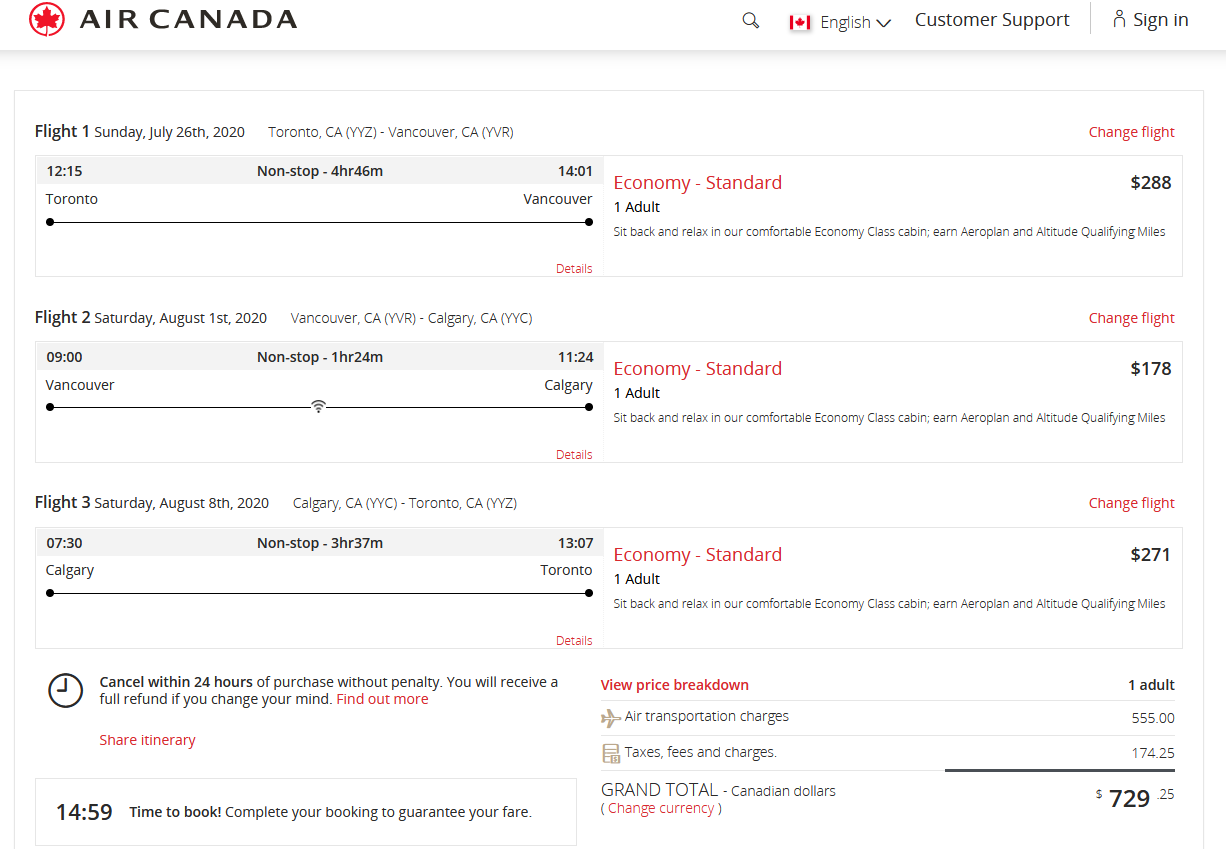The image depicts the Air Canada website interface. Prominently displayed in the top left corner are the Air Canada name and logo. On the top right corner of the screen, there are icons and links for search, language settings, customer support, and user sign-in. 

Below the header is a fine grey panel, leading to a rectangular section showcasing flight details. Each flight is detailed with its specific date, route, duration, and price, organized as follows:

1. **Flight 1**: A non-stop flight from Toronto to Vancouver, scheduled for Sunday, July 26th, 2020. The flight duration is 4 hours and 46 minutes, and the ticket price for one adult in Economy Standard class is $288.
   
2. **Flight 2**: A flight from Vancouver to Calgary on Saturday, August 1st, 2020. The flight lasts 1 hour and 24 minutes, with a ticket cost of $178 for one adult in Economy Standard class.

3. **Flight 3**: Scheduled for Saturday, August 8th, 2020, this flight travels from Calgary to Toronto. The flight duration is 3 hours and 50 minutes, with the ticket priced at $271 for one adult in Economy Standard class.

Each flight's pricing is displayed on the right side of the section in red text, with a total combined cost amounting to $729.25 for all three flights.